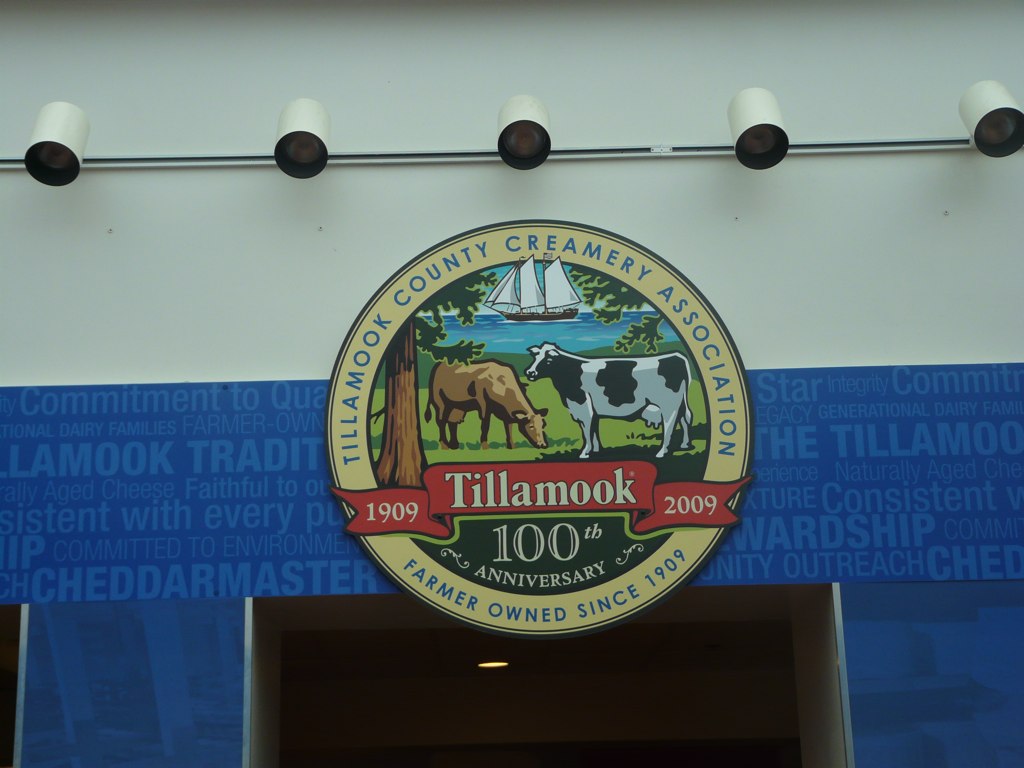This image features a detailed sign advertising the Tillamook County Creamery Association, celebrating its 100th anniversary. Central to the sign is a logo depicting two female cows eating grass, one of which is brown and the other is the classic black and white spotted. Surrounding the cows, in a circular arrangement, are the words "Tillamook County Creamery Association, 1909 Tillamook, 2009, 100th Anniversary" and at the bottom, "Farmer Owned Since 1909." 

The logo sits on a white wall beneath five downward-pointing lights. Behind the logo is a blue tarp adorned with the company's slogans such as "Tillamook Tradition," "Consistent Stewardship," "Outreach," and "Cheddar Masters." Below the logo, there is a doorway. The overall setting suggests a proud display of the company's heritage and commitment to quality.